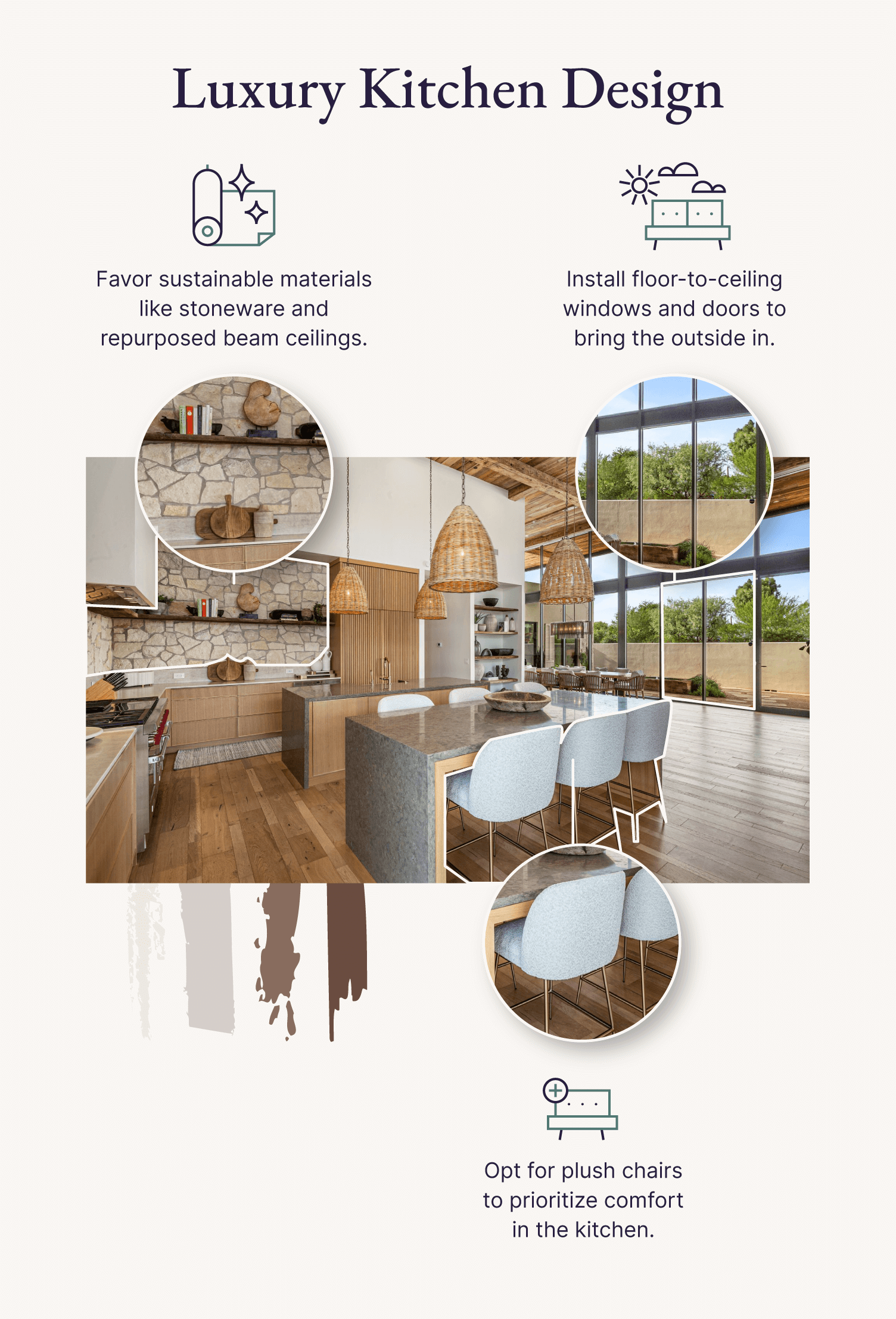This meticulously crafted infographic advertises a luxury kitchen design. The title at the top of the image is presented in black text against an off-white background, reminiscent of sophisticated wall paint. On the left, there's an icon resembling a roll of wall covering promoting the use of sustainable materials like stoneware and repurposed beam ceilings. A complementary icon on the right features a sun with clouds and suggests installing floor-to-ceiling windows and doors to seamlessly merge indoor and outdoor spaces. Additionally, the lower right corner highlights an option for push or plush chairs, emphasizing comfort in the kitchen.

In the center of the image, an interior shot reveals a beautifully designed kitchen with hardwood floors and a rustic yet modern appearance. The kitchen includes large windows and a glass door, offering ample natural light. The space features white-painted walls and a unique rock arrangement on the left, contrasted by wooden beams on the ceiling. A central countertop anchors the room, surrounded by six sleek, futuristic white chairs, positioned around a dining table. Hanging lights add a touch of elegance, enhancing both the functionality and aesthetic of the space.